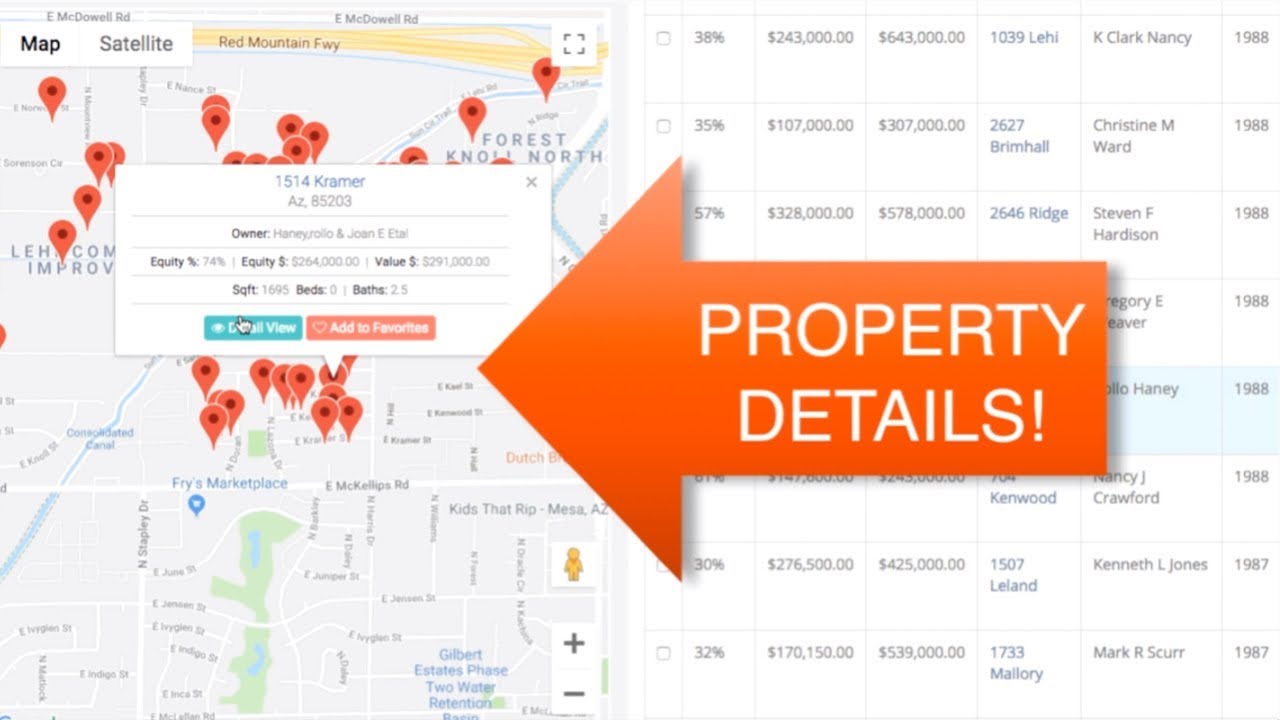The image displays a detailed layout, split into two main sections. On the left side, there's a map of a city. The map is labeled with "map" and "satellite" options in the top left corner. Centered on the map is a popup that shows an address, information about the owner, and two actionable buttons: "View" in blue and "Add to Favorites" in red. The map is adorned with numerous red icons, particularly concentrated at the top and around the center.

Directly in the middle of the image, an imposing orange arrow spans across the divide, pointing left. The arrow bears the text "Property Details" in bold white letters.

To the right of the arrow, the image contains a structured column of property information. This data is organized into 8 horizontal rows, with each row corresponding to an individual property. Each row includes several details: a percentage value, two prices (a smaller price followed by a larger price), an address with a house number, the owner's name, and the year the property was built. The background of this right-hand section is a light gray color, which matches the light gray hue covering most of the map area on the left.

Overall, the design is clean and data-rich, providing a clear snapshot of property details juxtaposed with geographic context.